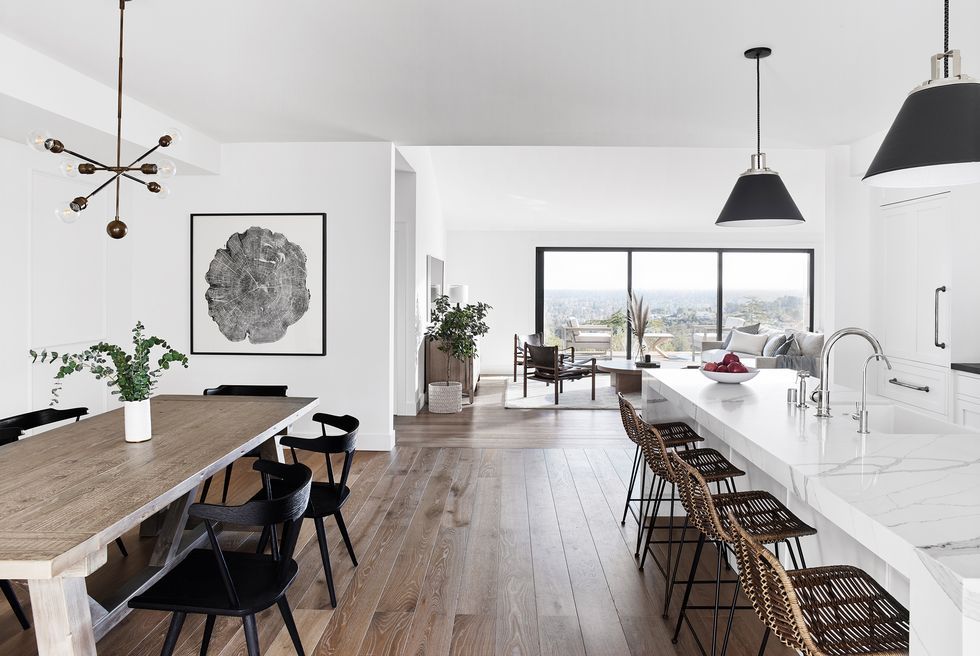This image captures the open-concept main floor of a large, modern home, combining kitchen, dining, and living areas. The space is characterized by its clean, contemporary design with white walls and brown wooden floors. In the foreground to the right is the kitchen, featuring a large white marble island equipped with a stainless steel sink and faucet. The island is accessorized with a white bowl filled with apples and surrounded by four wicker stools.

On the left side of the foreground is the dining area, anchored by a light wooden table surrounded by basic black wooden chairs. A modern, artistic pendant light, reminiscent of an atom, hangs above the table. The table itself is topped with a white vase containing a green plant. A prominent piece of art, depicting the cross-section of a tree trunk, adorns the adjacent wall.

In the background, the living area extends the open layout, with matching white walls and light wood furniture. It features a couch, a coffee table, and additional seating, all arranged to make the most of the large glass windows or sliding doors that allow for a stunning view of the cityscape outside. The space also includes a few green potted plants, enhancing the room's fresh and organic feel.

The design elements, from the white marble countertops to the black-framed windows, combine to create a harmonious and expansive living space that is both functional and aesthetically pleasing.